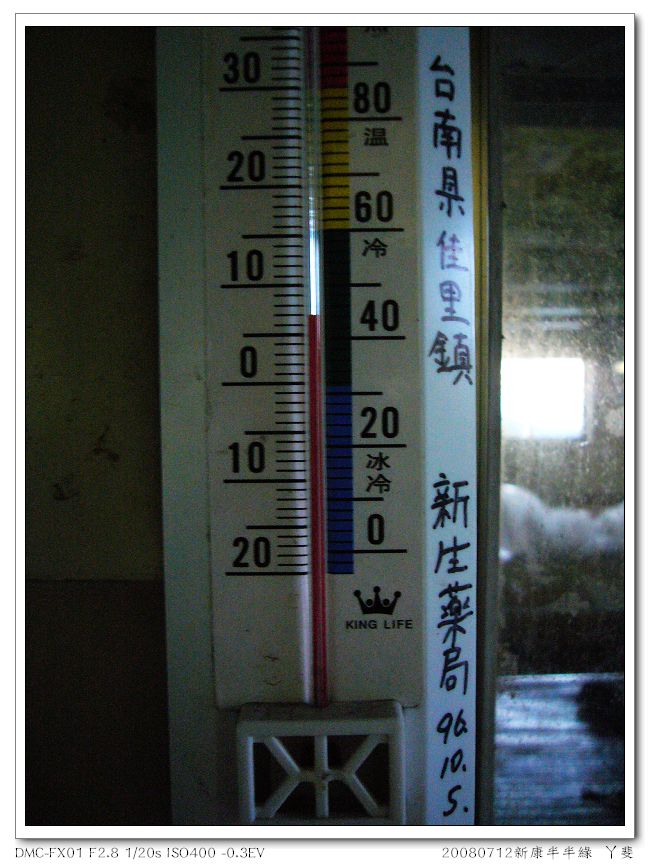This photograph, bordered by a thin white edge, presents a slightly grainy appearance. Underneath the image, there are gray numbers, letters, and some foreign-looking symbols. The central subject of the photograph is a white thermometer, prominently featuring foreign symbols reminiscent of Japanese or Chinese characters along its edge in black font. The thermometer displays its readings with black numbers, while its brand, "King Life," is marked in black above a black crown icon. A striking red stripe runs mid-center through the thermometer.

On one side of the thermometer, the numbers are in plain black with accompanying dash marks indicating measurements. On the opposite side, black numbers are interspersed with colored bars: starting from the bottom with blue bars, then a green bar, followed by a yellow bar, and culminating in a red bar at the top, denoting varying temperature ranges.

The background reveals a partial view of a mirror, reflecting a window through which sunlight streams. The wall behind the thermometer appears worn, showing visible black dirt and scuff marks. The mirror’s reflection captures the sunlight filtering in, adding an element of natural light to the scene.